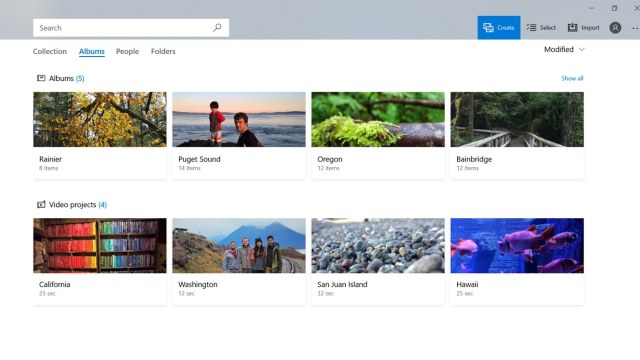The image appears to be a screenshot of a photo management webpage, showcasing a user's organized collection of photograph albums and video projects. On the left-hand side, there is a navigation panel with options labeled "Albums," "Collection Albums," "People," and "Folders," along with a search bar positioned above these categories. The "Albums" section contains five distinct titles: "Rainier" with approximately eight photos, "Puget Sound" with around 14 photos, "Oregon" with 12 photos, "Bainbridge" (appearing to be correctly named) with 12 photos, and a generic "Video Projects" category.

Within the "Video Projects" section, there are four subcategories listed as "California," "Washington," "San Juan Island," and "Hawaii." Each subcategory name is followed by a number that presumably refers to the video's duration in seconds: "California" with 25 seconds, "Washington" with 12 seconds, "San Juan Island" with 32 seconds, and "Hawaii" with 25 seconds. In the upper right-hand corner of the interface, there are buttons labeled "Create," "Select," and "Import" alongside a small profile icon. Below these buttons, options labeled "Modify" and "Show All" are visible.